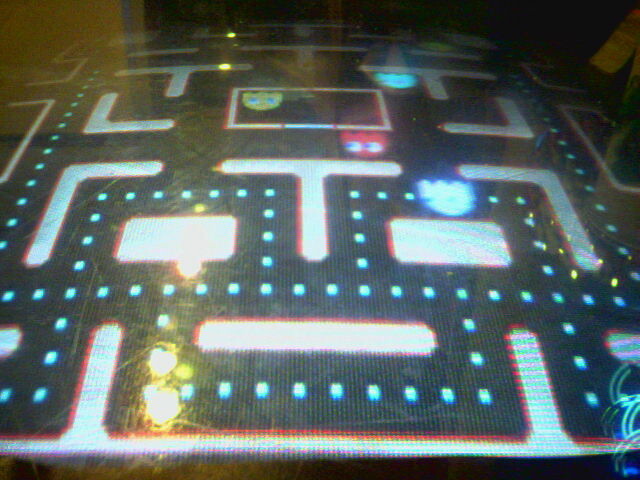The image is a detailed close-up of an old arcade machine screen displaying the classic Pac-Man game. The screen is viewed from a slight angle, giving a sense of depth and perspective. The black background is interspersed with white lines forming a maze pattern dotted with small blue pellets, which represent the food Pac-Man eats. Various L-shaped white barriers are visible throughout the maze.

At the top of the screen, the characters appear upside down due to the viewing angle. There's a red ghost with blue eyes, a light blue ghost, a yellow ghost, and what appears to be a white ghost with a crown above it. In the center of the screen, Pac-Man, a yellow circular creature with blue eyes, is positioned within a white box segment of the maze. The bottom edging of the screen is black, contributing to the overall dark aesthetic. 

Additionally, the image captures the nostalgic essence of the arcade machine; there are visible scratches on the glass and reflections of lights, particularly noticeable in the bottom right corner. This adds a layer of authenticity and wear, as if the machine has been well-used over the years.